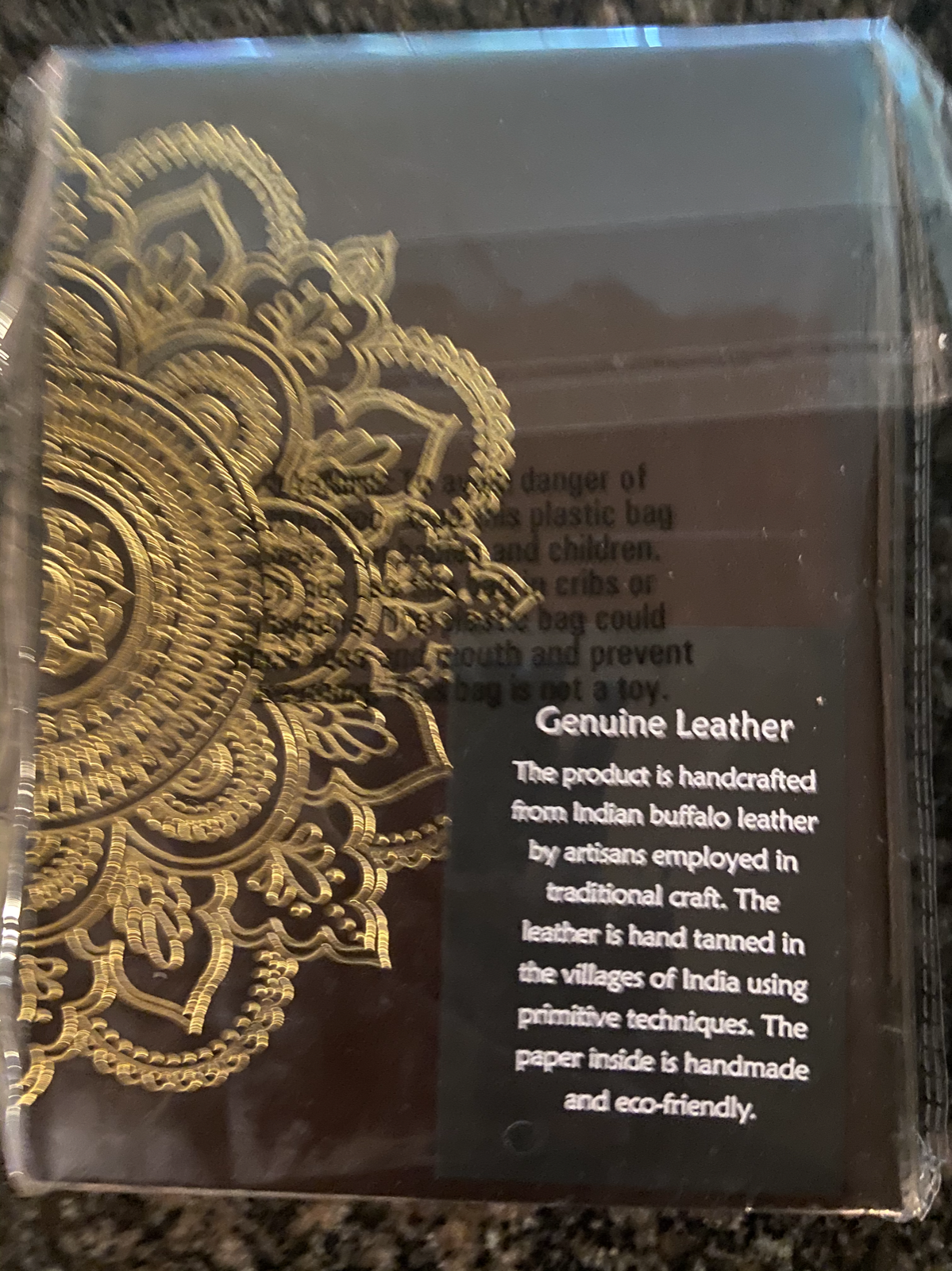The photograph showcases a handcrafted book made from genuine Indian buffalo leather. The book, encased in a shiny plastic sleeve for protection, prominently features a large gold flower design on its rich brown leather cover. In the foreground, the image captures a countertop, possibly granite, in shades of black, brown, and tan, providing a contrasting background. The packaging includes a visible warning about the dangers of plastic bags around children. There is also a black tag or sticker on the book that states in white text: "Genuine Leather. This product is handcrafted from Indian buffalo leather by artisans employed in traditional craft. The leather is hand-tanned in the villages of India using primitive techniques. The paper inside is handmade and eco-friendly."